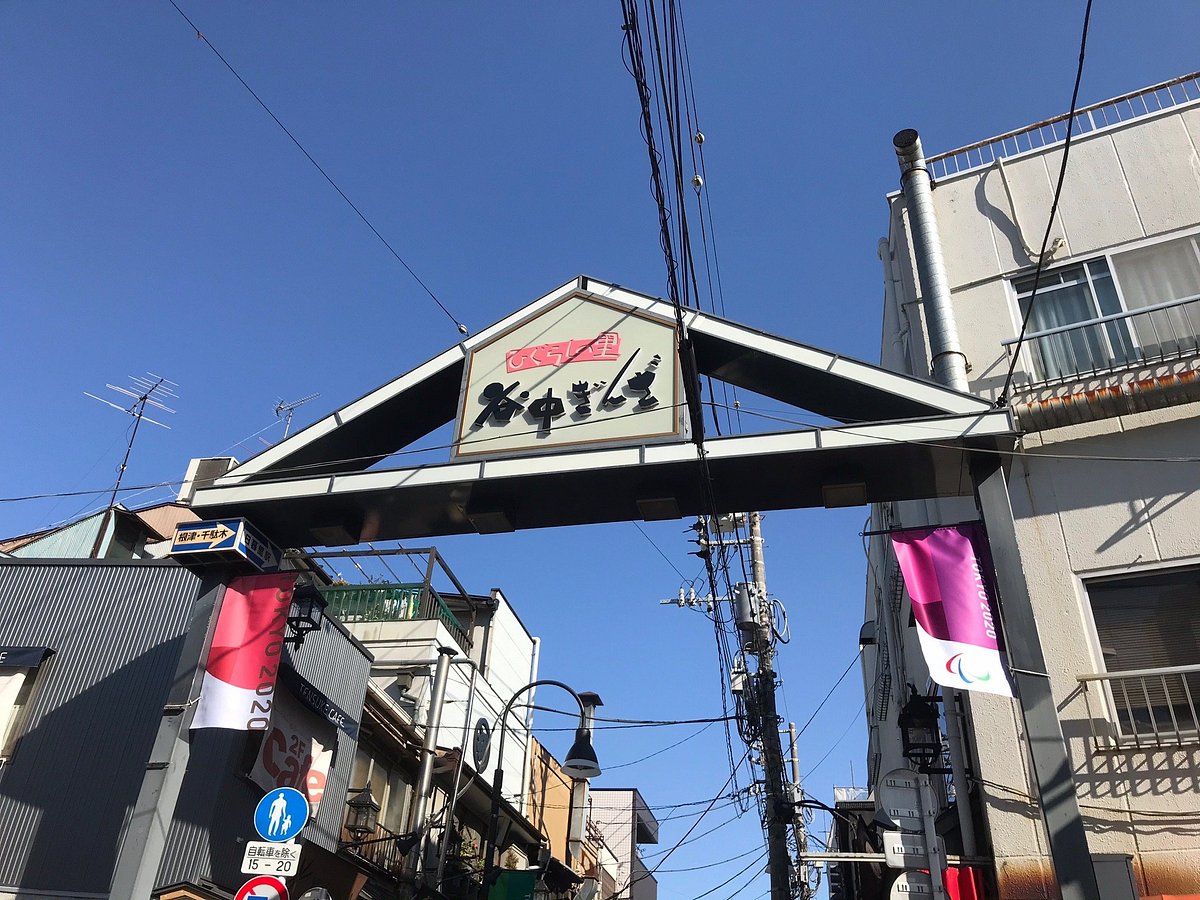This color photograph captures an urban scene with a clear blue sky occupying most of the upper part of the image, emphasizing the wild web of electrical wires strung high above. The camera is angled slightly upwards, revealing a densely populated array of wires, cables, and antennas stretching across and connecting various points. These lines converge dramatically around a triangular arch that bridges two buildings on either side of a bustling shopping area. This arch, adorned with Asian characters—likely Korean or Japanese—serves as a focal point, emphasizing the chaotic tangle of lines that pass through it.

On the right, a two-story cement building features balconies with metal fences and several windows, standing adjacent to a taller, white, three-story structure. To the left, another building, gray in color, stands alongside a white building further along the street. Old-fashioned TV antennas are visible atop these structures, adding to the visual clutter of modern civilization.

Amidst these buildings and wires, a streetlight with a hooked design and a blue sign depicting white silhouettes of a person walking with a child marked "15 to 20" can be seen. The sheer volume of power lines, twisted and tangled, lends a hazardous appearance, reminiscent of urban scenes in cities like Bangkok, known for their dense, intricate networks of overhead wiring. The image vividly conveys the chaotic complexity and potential dangers of urban electrical infrastructure in an overseas cityscape.